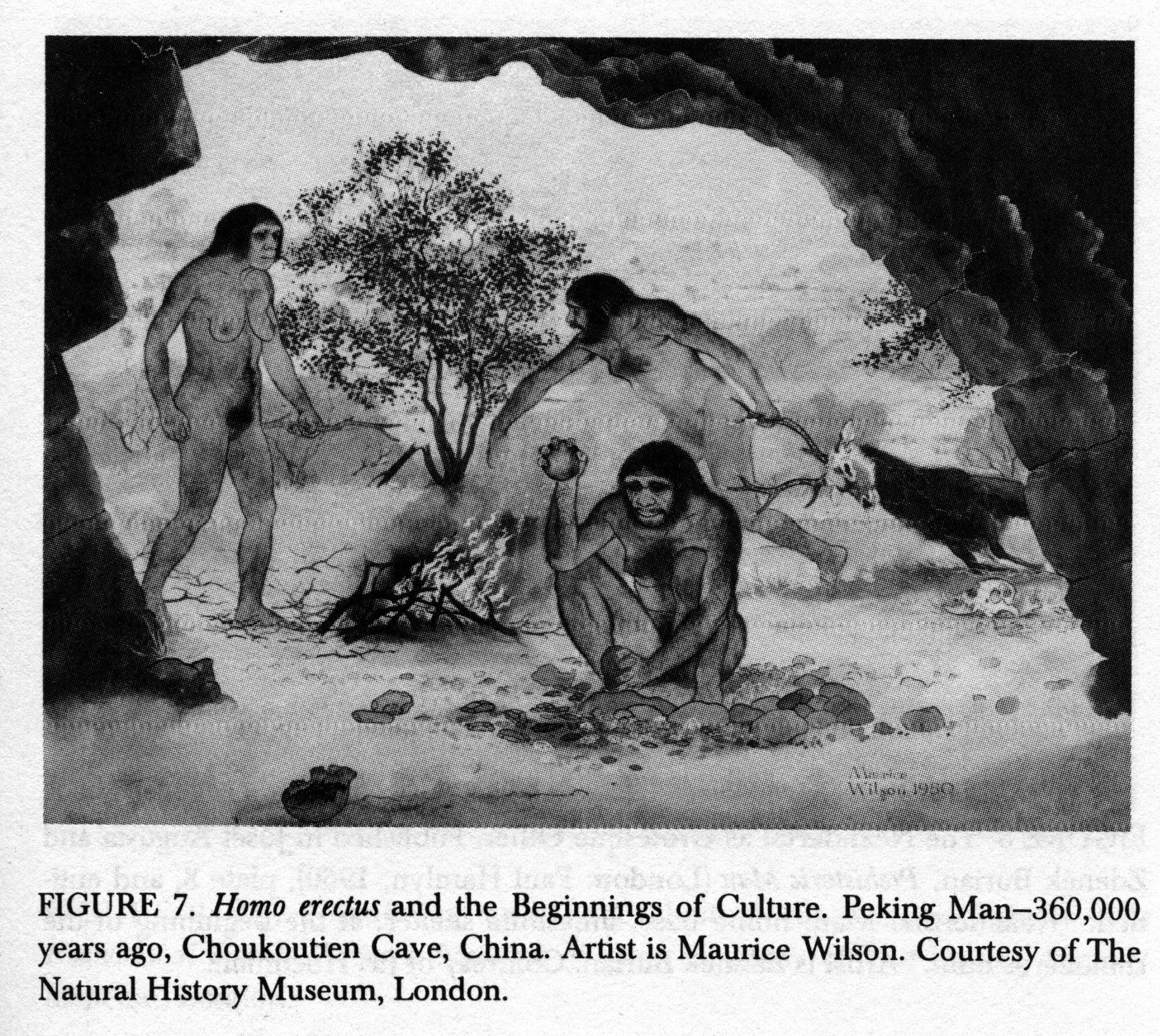The black-and-white image, likely from an old textbook or magazine, depicts an ancient scene titled "Figure 7: Homo Erectus and the Beginnings of Culture, Peking Man, 36,000 years ago, Chukotian Cave, China," drawn by Maurice Wilson and courtesy of the Natural History Museum, London. The detailed drawing, in pencil or charcoal, shows three cave-dwelling individuals—two men and a woman—engaged in early cultural activities. On the left, a woman, identifiable from her breasts, walks towards a fire with a stick in her hand. In the center, a man is kneeling amidst rocks, striking one rock with another, possibly attempting to create fire. Another man, positioned towards the left, drags a dead deer by its antlers. Behind them, a tree stands near the cave's entrance, with the cave walls arching around the scene from above. The background reveals an outdoor area, effectively capturing a moment in prehistoric daily life.